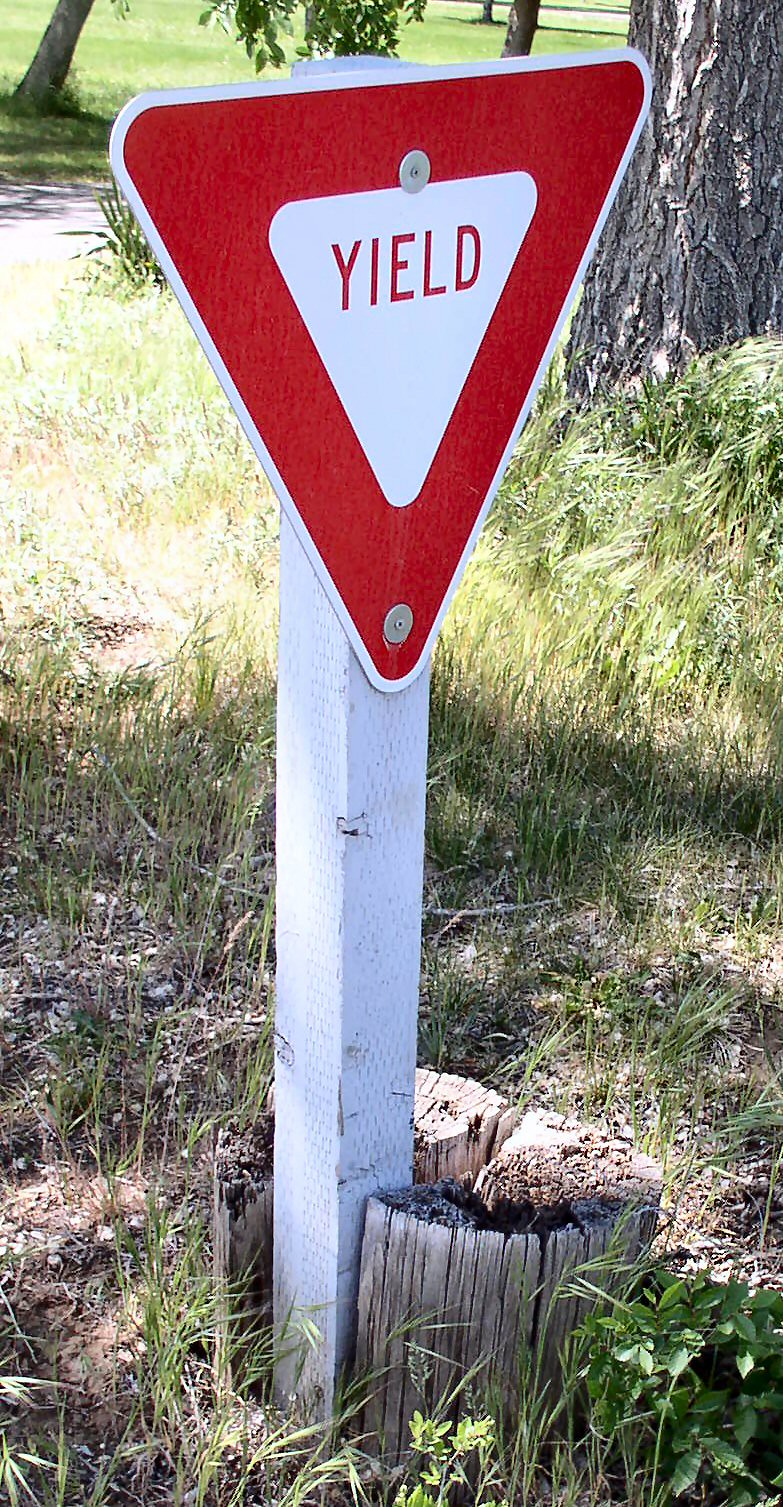The image depicts a short yield sign with a distinct triangular shape featuring a thick red border and a white interior with the word "yield" written in red. The sign is securely fastened with two metal screws onto a white-painted wooden post. This post is set into a section of an old tree trunk, which appears chopped down and blackened on one end. The area surrounding the sign is characterized by tall, unkempt grass, with patches of dry dirt and rocks visible. To the right of the sign, there's a dark, rough-looking tree trunk with patches of beige where the bark seems to have rubbed off. On the left, the grass is highlighted by sunlight, giving it a whitish appearance. In the background, there are additional green grassy areas and another tree whose trunk and lush leaves partly frame the view, along with what seems to be a road or driveway extending into the distance.